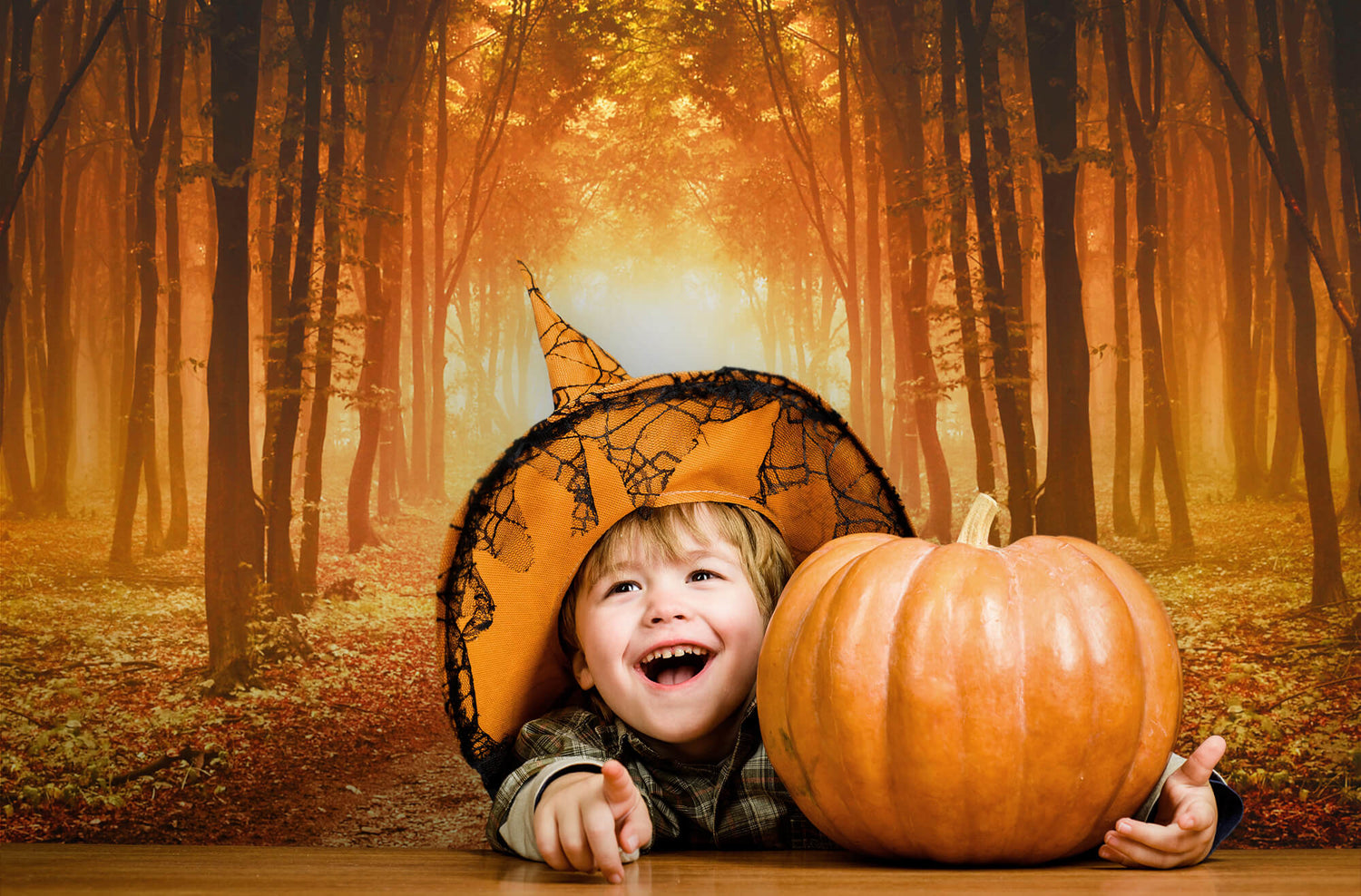This photograph captures a joyous young boy seated at a brown wooden table in an enchanting autumn setting. The child, a white boy with short blonde hair, exudes happiness as he smiles broadly, revealing his teeth, and points upwards with his right index finger. He dons an orange witch's hat adorned with black webbing along the brim, perfectly complementing his brown flannel shirt. With his left arm wrapped affectionately around a large, shiny, uncarved orange pumpkin, he adds to the festive atmosphere. The backdrop resembles a canvas print depicting a picturesque fall scene: a dense forest with tall, dark trees and fallen orange leaves blanketing the ground, illuminated by the warm, amber glow of a setting sun. The composition suggests a Halloween-themed portrait set in a magical woodland, evoking the essence of the autumn season.